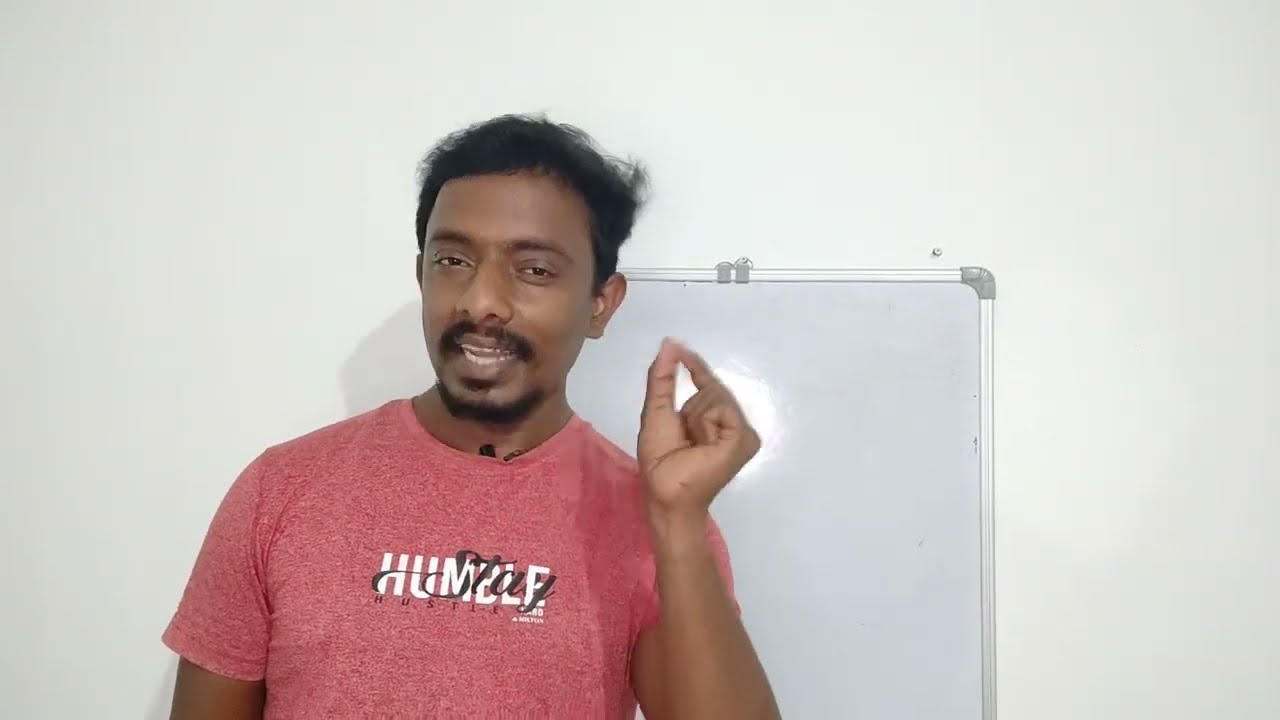In the center of this horizontally oriented image is an Indian man with brown skin, standing in front of a vertical whiteboard framed in thin silver metal, mounted on a white wall. The man has frizzy, somewhat unkempt black hair, brown eyes, and a brown beard and mustache. He is wearing a red t-shirt that reads "stay humble" and possibly "hustle" in white and black lettering. His right arm is down, while his left arm is bent at the elbow, with his hand raised parallel to his cheek, thumb and forefinger pressed together as if he is snapping his fingers. The man appears to be in mid-conversation, his mouth slightly open, conveying an expression of making a point or perhaps saying something humorous. There are no writings or markers visible on the whiteboard behind him.